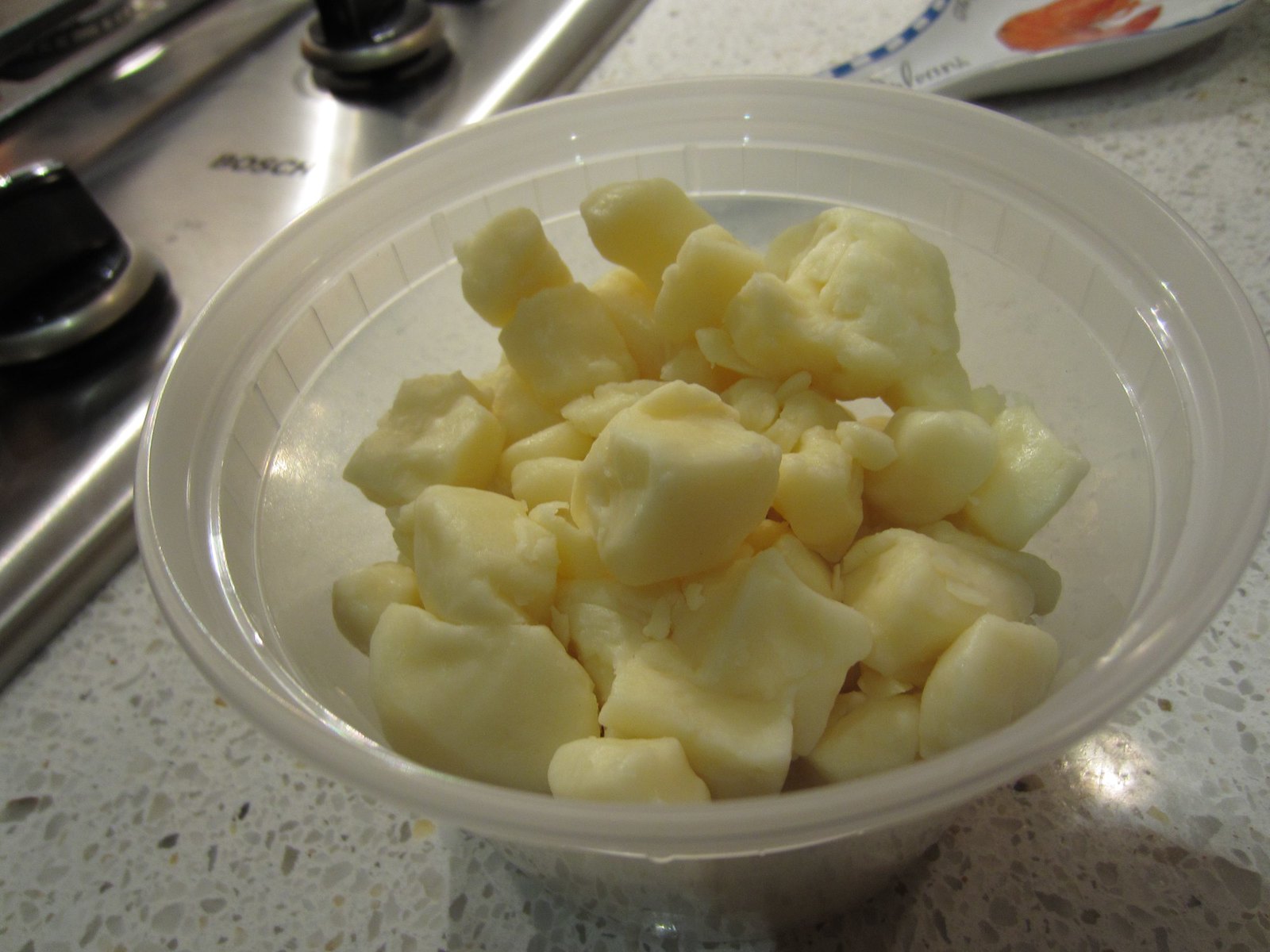This photograph captures a cozy kitchen scene centered around a meal preparation in progress. At the heart of the image is a transparent, fluted plastic bowl, about three-quarters full with numerous yellowish white lumps of what appear to be cheese curds. The cheese curds, often referred to as "squeaky cheese" due to their unique texture, are irregular in size and shape, corresponding with typical cheese curd characteristics. The bowl rests on a pristine, speckled countertop, likely made of granite or laminate, in shades of gray, beige, and black. Behind the bowl, a sleek silver BOSCH oven with various knobs is visible, adding a modern touch to the setting. To the left of the bowl, a glass spoon holder subtly complements the kitchen's organized ambiance. The detailed and tactile elements in the composition evoke a sense of homeliness and culinary anticipation.